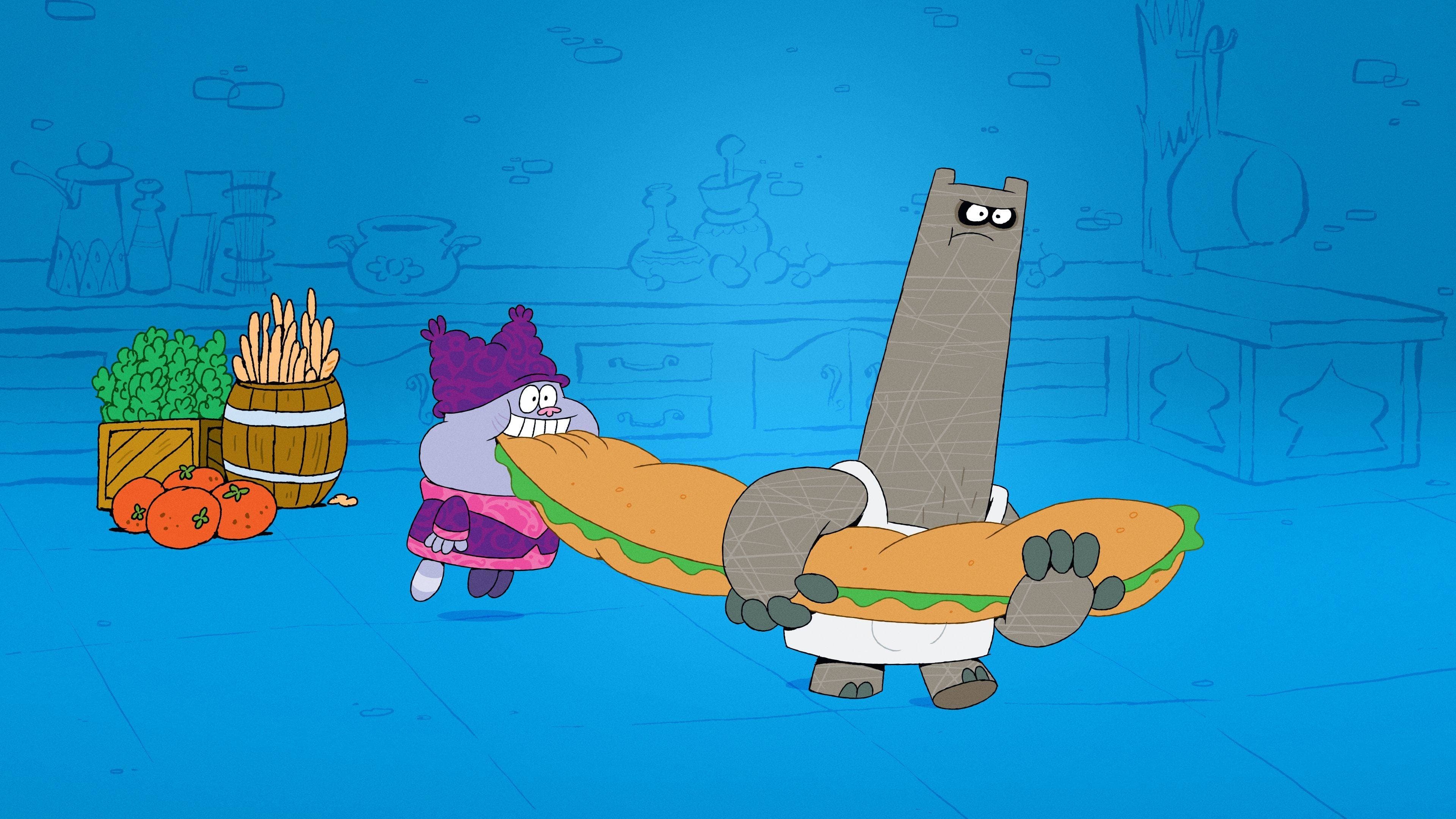The image is a vibrant cartoon scene, likely from the animated show "Chowder," set in what appears to be a kitchen. The background is uniformly bright blue with minimal detail, resembling a blueprint sketch of kitchen elements such as cabinets, drawers, and countertops, which stretch across the scene. In the kitchen, there are various objects such as a teapot, cooking pots, and a hanging pot. On the left side, a crate filled with green leaves and a brown barrel, possibly containing long breadsticks or sub-rolls, are visibly more detailed. In front of this setup, four large, vividly red tomatoes are scattered on the floor.

Dominating the foreground are two colorful characters engaged in a comedic moment. On the right is Schnitzel, a tall, gray, hulking creature with a block-like elongated neck and dark black eyes, wearing a white tunic. He is carrying a comically oversized submarine sandwich, with green lettuce poking out between the slices of brown bread. Trailing behind him, Chowder, the smaller and round-faced character with light purple skin, is floating in mid-air. His large white teeth are clamped onto the back end of the sandwich. Chowder is adorned in a distinctive purple hat and a matching outfit that includes a purple and pink jacket, completing the whimsical scene.